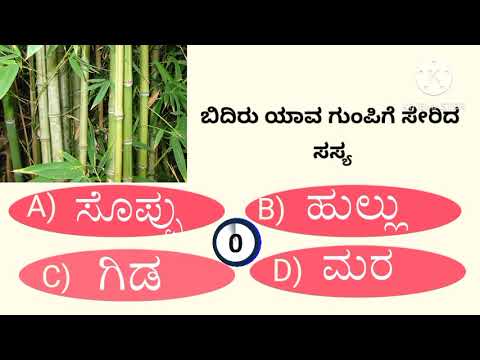The image depicts what appears to be an interactive ad or a question-and-answer interface in a foreign language. It features a black border at the top and bottom, with a peach-colored background in between. In the upper left corner, beneath the top border, there is a close-up image of green bamboo plants. To the right of this image, there are black letters or symbols with a small logo above them. The main focal point consists of four red, capsule-shaped buttons labeled A, B, C, and D, each containing unknown foreign text. In the center of these buttons is a circle displaying the number zero, suggesting a timer or score count. The entire image is vibrant and well-defined, resembling a game show or quiz interface where users choose from multiple-choice answers.